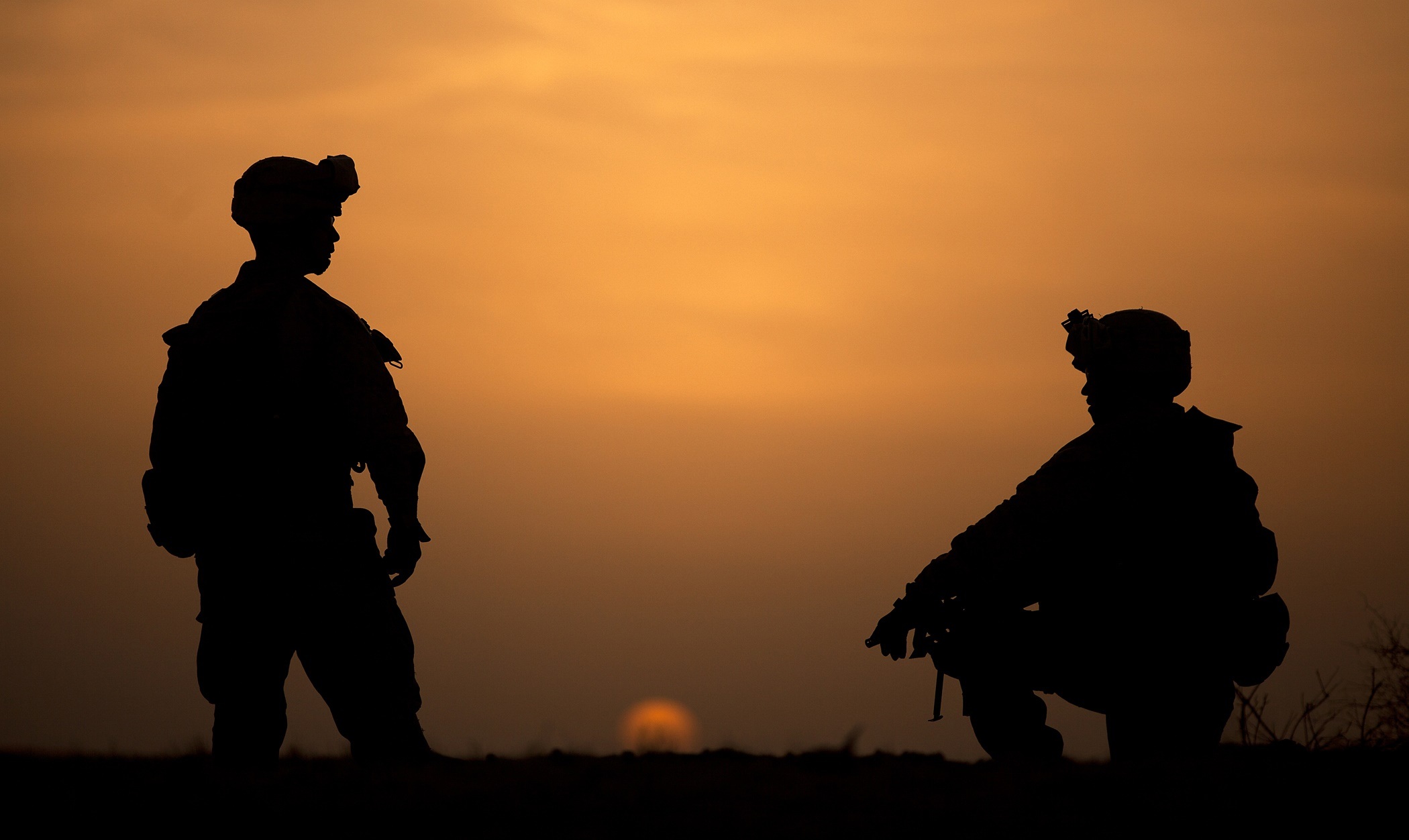In this professionally staged full-color photograph taken at sunset, two soldiers are silhouetted against a dramatic sky painted with hues of gold, orange, and red. The sun, positioned just at the bottom of the horizon, casts a dim but striking glow. The soldier on the left stands upright, his head turned towards the kneeling soldier on the right. Both are dressed in full army uniforms, complete with helmets and night vision goggles. The soldier on the left's silhouette reveals equipment strapped to his body, while the soldier on the right, kneeling on his right knee with his left foot firmly planted on the ground, braces a rifle across his knee. Small scrub plants can be seen faintly behind the kneeling soldier, adding a touch of natural detail to the scene. The sky, covered in heavy clouds, amplifies the poignancy of the sunset and the solemnity of the moment between the two soldiers.